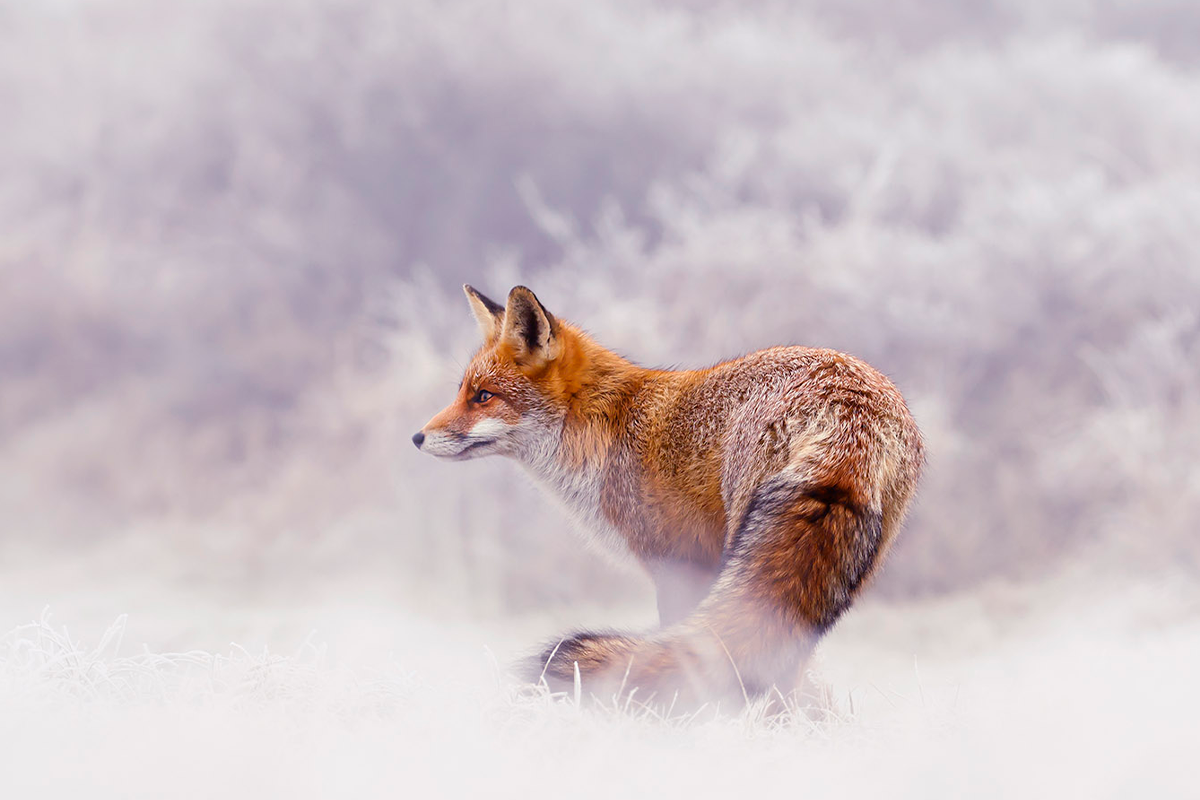The image features a beautiful red-tailed fox standing prominently against a predominantly white background that resembles snowy clouds, interspersed with slight hints of purple. The fox, primarily a rich reddish-brown with patches of white under its chin, throat, and along its whisker area, is captured from a backside angle, giving a clear view of its curved back and fluffy, black-tipped tail partially concealed by the white background. The fox's ears are pointed straight up, and its golden eyes are intently gazing to the left, suggesting that it is alert and focused on something out of the frame. Although the overall scenery is dominated by white, a few grass blades and bushes slightly frosted can be discerned in the background, enhancing the natural setting. The fox appears healthy and robust, a striking presence within the serene, almost surreal landscape.